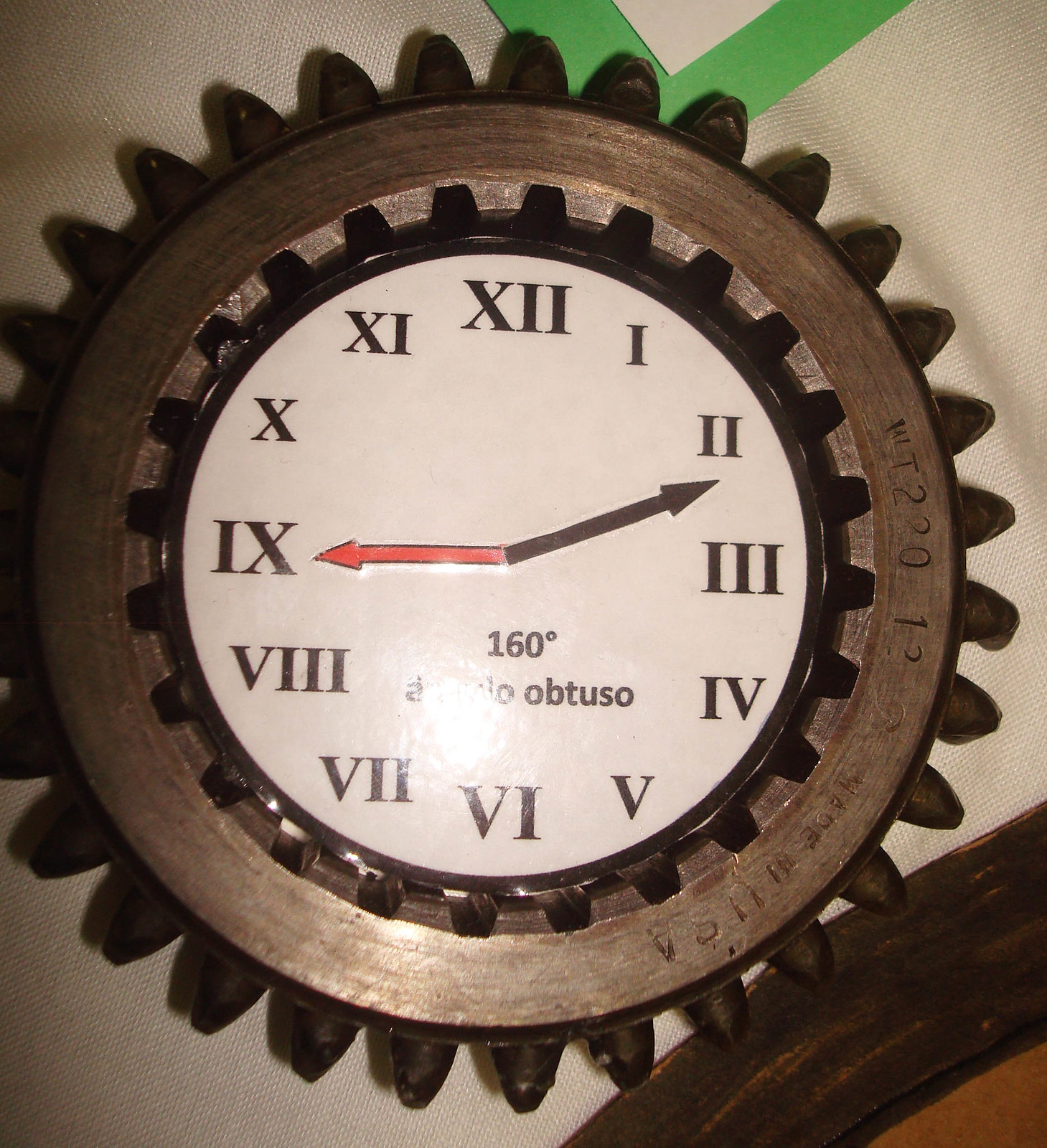This image features a distinctive clock with two gear-like wheels, located against a whitish cream fabric background, reminiscent of a couch cushion. The clock exhibits an outer wooden gear with brown rivets along its black or brown outlined edges. There is an additional smaller wooden gear within the center. Both gears are surrounded by intricate metalwork, suggesting a blend of rustic and industrial design styles. Roman numerals from I to XII mark the hours on the clock face. The clock's hour hand points to IX (9), while the minute hand is situated between II (2) and III (3), indicating a time of approximately 2:45. Below the center, in black lettering, the inscription reads "160 degrees angulo obtuso," with another word "Abtuso" partially visible. Above the clock, a hint of green is seen, possibly from a plant, and in the bottom right corner of the image, a reddish-brown circular wooden frame or object is partially displayed.